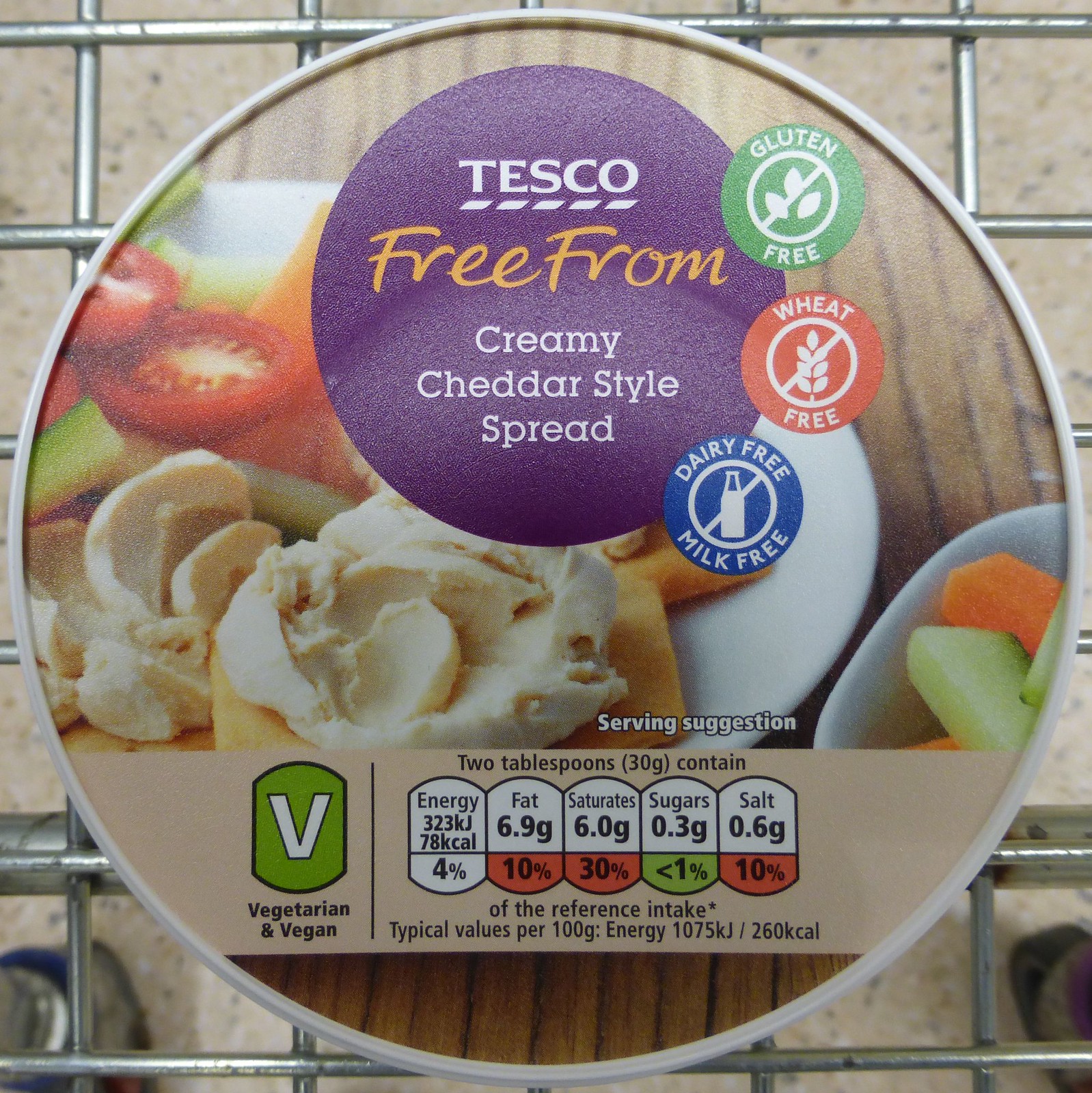The image depicts a circular container of cheese spread, specifically Tesco's "Free From" Creamy Cheddar Style Spread, placed in a grocery cart with a metallic grid background. The container features a visually striking lid design, dominated by a deep purple circle with "Tesco" written in white font, followed by "Free From" in orange, and "Creamy Cheddar Style Spread" in white. Adjacent to this, three smaller circles convey key dietary information: a green circle proclaiming "Gluten Free," an orange circle stating "Wheat Free," and a blue circle noting "Dairy Free, Milk Free," each with corresponding icons.

The lower part of the lid includes a beige banner presenting nutritional information and dietary tags. A bright green shield with a white "V" indicates the spread is suitable for vegetarians and vegans. The banner details the nutritional content per two tablespoons (30g): 323 KJ/78 Kcal of energy, 6.9g of fat, 6.0g of saturates, 0.3g of sugar, and 0.6g of salt. These values are accompanied by percentage intake figures, color-coded for clarity.

In the background of these elements, the lid's design features a rustic wooden table with a white plate and a bowl filled with an assortment of colorful vegetables and crackers topped with the cheese spread, visually emphasizing possible serving suggestions. This combination of detailed dietary information and appealing visual cues aims to inform and attract health-conscious consumers.